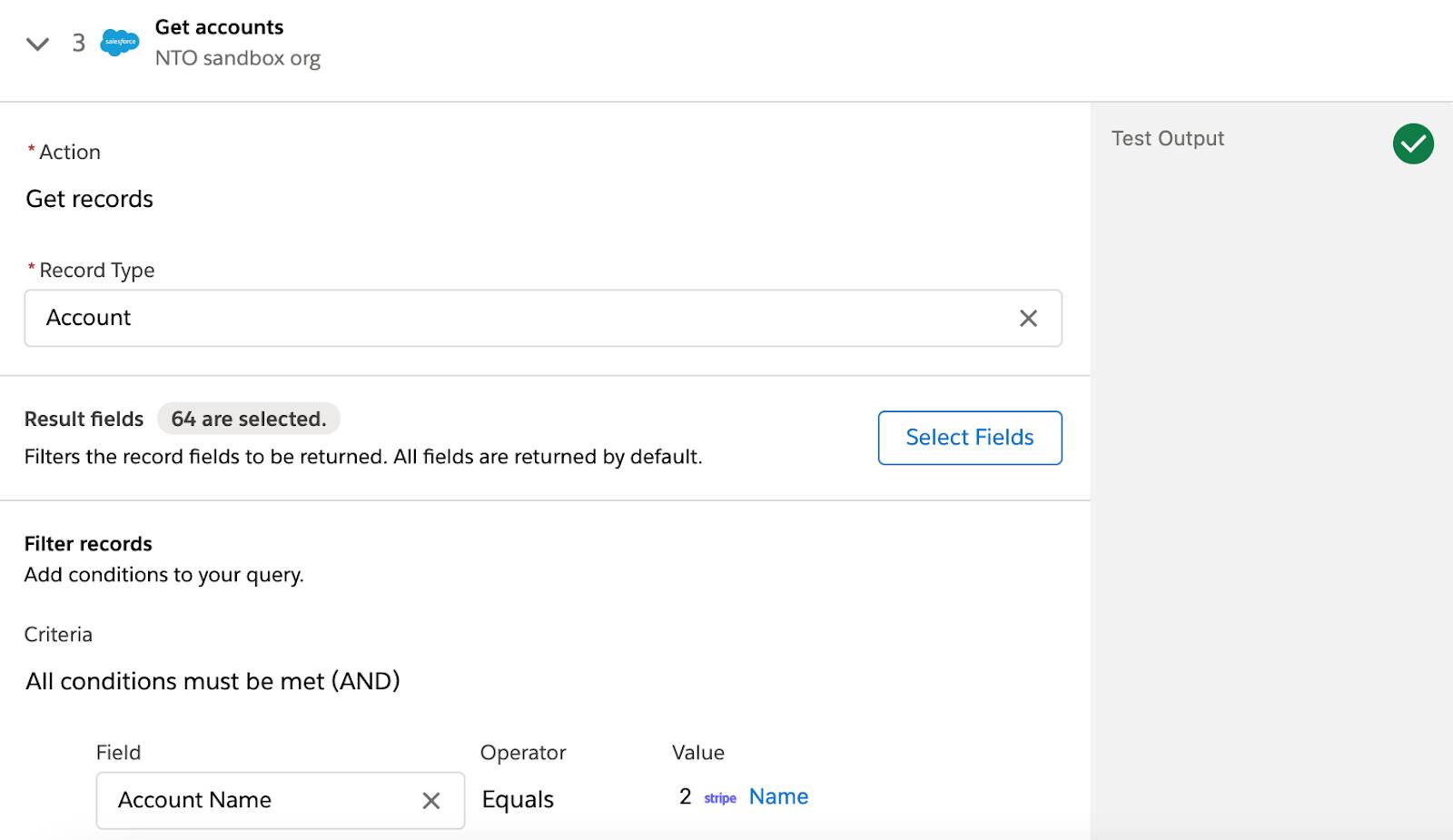A computer screen displays an interface with a number of elements related to Salesforce. At the very top left corner, there is a "Number 3" accompanied by a down arrow. Next to it, a bluish-teal bubble icon resembling a cloud bears the word "Salesforce." Adjacent to this icon, the text "Get Accounts" is prominently displayed in bold, with "NTO Sandbox Org" in smaller grey text underneath.

A dividing line separates the top section from the rest of the content below. On the far right side, there is a skinny grey rectangle featuring a green circle with a white check mark inside it. Above this circle, the words "Test Output" are written at the top of the rectangle.

On the left side of the screen, the content continues with the header "Action" followed by the subheader "Get Records." Further down, it reads "Record Type" with "Account" beside it, along with a field for user input. Below this, it states "Result Fields" with a note that 64 fields are selected. An area titled "Filters" indicates that "All fields are returned by default." There is also a clickable blue button labeled "Select Fields."

The page appears consistent in its formatting as the user scrolls further down, maintaining a structured layout for interacting with Salesforce data.